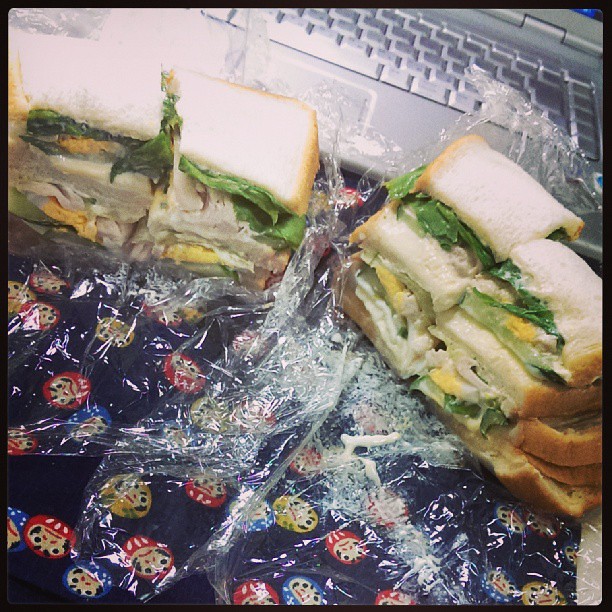The image depicts two partially unwrapped, triple-decker deli sandwiches positioned in front of a gray laptop keyboard, with the screen outside of the frame. The white bread sandwiches are layered with turkey, lettuce, and mustard, and there are hints of egg and possibly mayonnaise. The opened plastic wrap lies beneath and around the sandwiches. The ensemble rests on a dark blue tablecloth adorned with red, yellow, and blue faces.